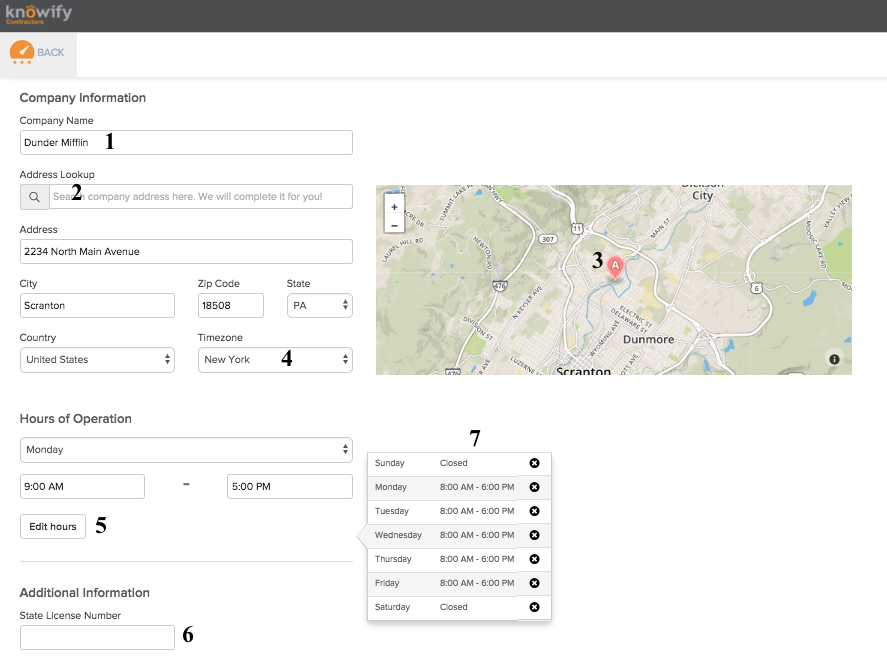This screenshot from the Knowify Contractors platform features the company information for a business named "Dunler Mifflin." Key details include:

1. **Company Name**: Dunler Mifflin
2. **Address Lookup**: (Box 2) - Empty
3. **Address**: 2234 North Main Avenue
4. **City**: Scranton
5. **Zip Code**: 18508
6. **State**: PA
7. **Country**: United States
8. **Time Zone**: New York (Box 4)

To the right of the address details, a map (Box 3) highlights the specific location with a marker. Additionally, the screenshot presents the hours of operation, displayed as follows:

- **Monday**: 8 or 9 AM to 5 PM
- **Edit Hours**: (Box 5)

A detailed list of hours for each day of the week (Sunday through Saturday) is provided in a separate box. Another section, marked with Box 6, is designated for additional information but remains empty. The number 7 appears above the hours section, and the map to the right gives a visual indicator of the general area of the address.

Overall, the image comprehensively lays out essential company information, contact details, operation hours, and location specifics in a structured manner.